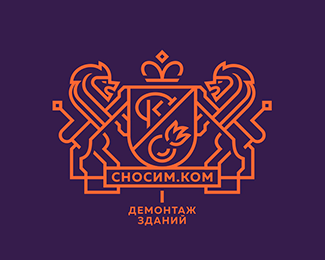The image depicts a modern, graphically designed crest set against a purple background. The crest is centrally positioned within a horizontal rectangle and highlighted by bold orange lines. On either side of the crest are two rudimentary, line-drawn lions standing on their hind legs with their paws raised, facing each other. The lion on the left faces right, and the lion on the right faces left, both appearing to support an orange-outlined shield in the center. The shield features a diagonal crossbar running from the bottom left to the upper right. Above the shield is a crown adorned with two arches, a horizontal bar, and a diamond outline at its peak. The upper section of the shield is marked by a symbol resembling a K with a circular line wrapping around its top. The lower section of the shield bears an image that might be a piece of fruit or a flower. Below the shield, a horizontal bar string features bold orange lettering in Cyrillic: "C-H-O-C-N-M dot K-O-M." Further down, a vertical bar extends to more orange Cyrillic text. The design melds traditional heraldic symbols with contemporary graphic elements, emphasizing a blend of historical and modern aesthetics.